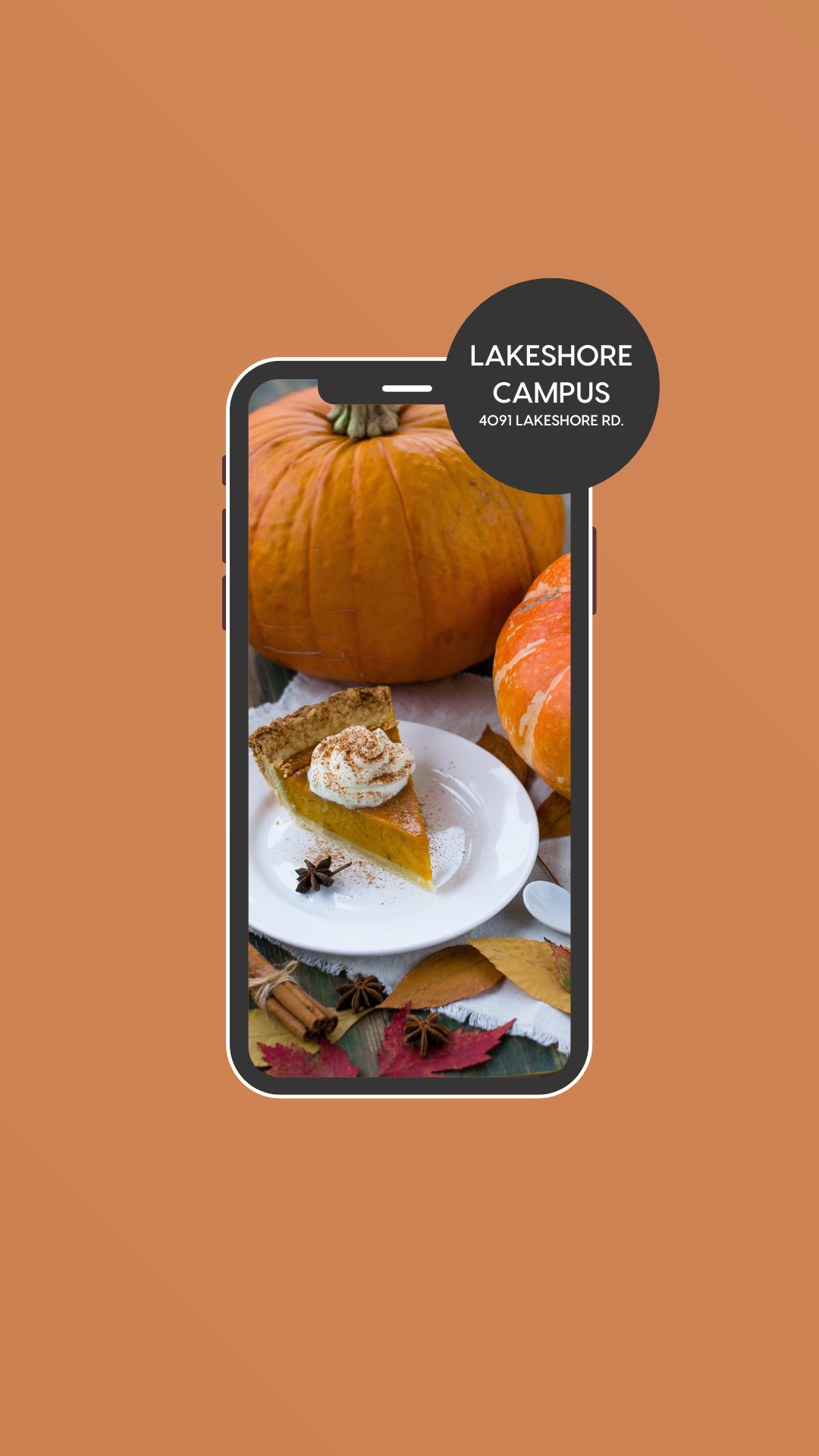In the image, a mobile phone screen displays a slice of pumpkin pie adorned with a swirl of whipped cream and a dusting of cinnamon. The phone is set against a festive autumnal background featuring two large, vibrant orange pumpkins. The tabletop holds rustic decorations including dried maple leaves, several cinnamon sticks tied with string, and cloves. On the corner of the mobile phone screen, a black circle contains the text "Lakeshore Campus, 4091 Lakeshore Road." The backdrop of the image showcases a warm, peachy orange hue, likely suggesting graphics promoting a Halloween party at Lakeshore Campus. This visually enticing scene implies an event celebrating Halloween, complete with sumptuous seasonal treats and festive decor.